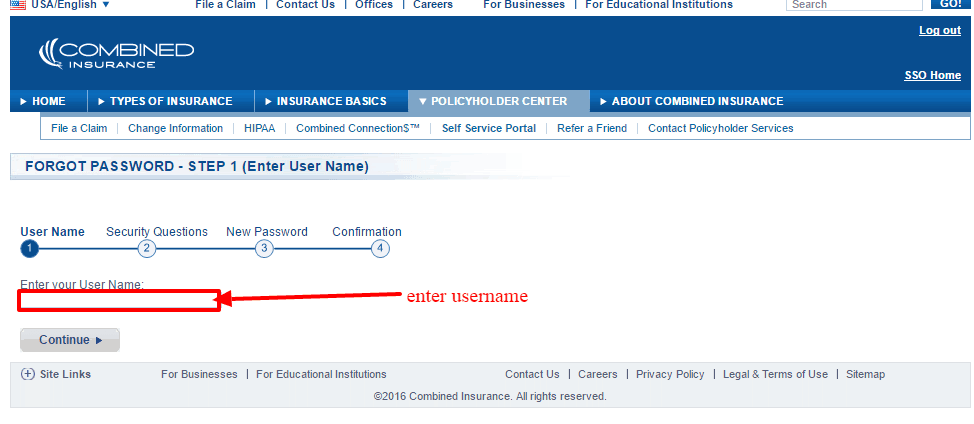This image is a screenshot of the Combined Insurance website, showcasing the header and several functional sections. At the top of the screen, it features the USA flag icon with the text "USA | English" and a drop-down menu. The menu includes options such as "File a Claim," "Contact Us," "Offices," "Careers," "For Business," and "For Educational Institutions." To the right side of the header, there's a search bar for easy navigation.

Below the header, a prominent banner displays the name "Combined Insurance." Under this banner, the navigation menu includes links to "Home," "Types of Insurance," "Insurance Basics," "Policyholder Center," "About Combined Insurance," "File a Claim," "Change Information," "HIPAA," "Combined Connections," "Self-Service Portal," "Refer a Friend," "Contact Policyholder Service."

Further down, the section titled "Forgot Password: Step One" guides users through the process of recovering their account. It lists four steps: 
1. Username
2. Security Questions
3. Password
4. Confirmation 

The field for entering the username is highlighted with a red box labeled "Enter Username," next to which is a "Continue" button. At the bottom of the screen, additional information is provided, although it is not specified. This detailed layout emphasizes the website’s user-friendly design and accessibility features.